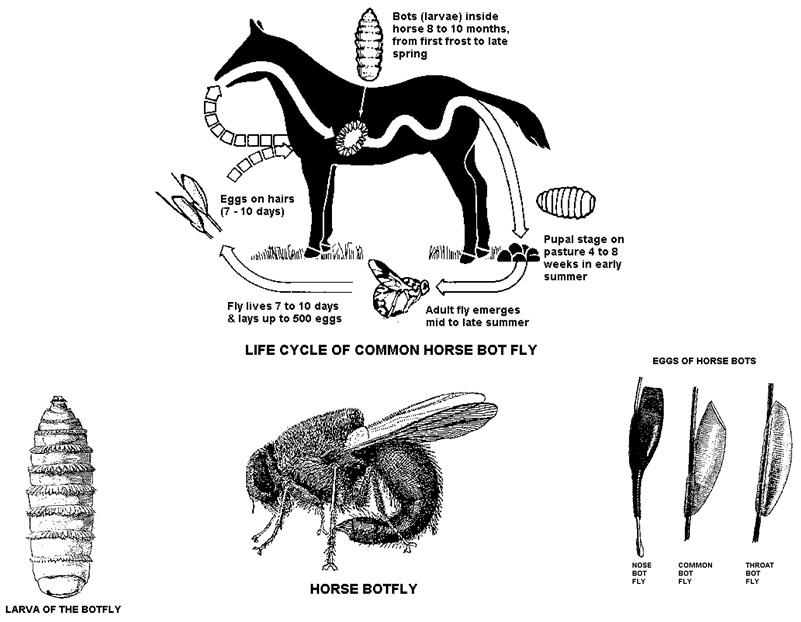This detailed black and white illustration depicts the life cycle of the common horse botfly (Gasterophilus). Central to the image is a horse, which is accompanied by labeled drawings and arrows explaining each stage of the botfly's life cycle. Above and behind the horse, there are illustrations of larvae, reinforcing the infestation process within the host. Below the horse, an adult fly is shown, representing the botfly's final stage.

Detailed annotations indicate that bot larvae reside inside the horse for 8 to 10 months, from the first frost to late spring. Arrows guide the eye from the horse’s mouth, through its digestive tract, and to its feces, visually explaining the larvae's journey. The larvae pupate in the pasture for 4 to 8 weeks during the early summer, subsequently emerging as adult flies mid to late summer.

Additional labels clarify that adult botflies have a lifespan of 7 to 10 days, during which a single fly can lay up to 500 eggs on the horse's hairs. To the right of the horse, the image includes drawings of these eggs, while the left side features an illustration of the larvae. The entire composition aims to provide an educational overview of botfly infestation in horses and is likely sourced from an academic or veterinary textbook.